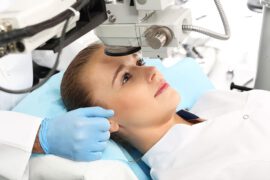The image is a small, low-resolution photo depicting a young woman lying on a reclining doctor's chair, fitted with a blue, sterile pillow. Her light brown hair is pulled back, and she is dressed in a white top, possibly a medical gown. Her face shows a neutral expression as she looks directly upward into a medical device positioned above her head. The device features a circular component over her eyes and has a silver knob near the top, along with a white body and a connected silver hose. A person, likely a doctor or technician, is partially visible behind her, identifiable by a white lab coat sleeve and a blue nitrile-gloved hand resting near her ear. The scene suggests that she is undergoing some form of medical imaging or scanning procedure.